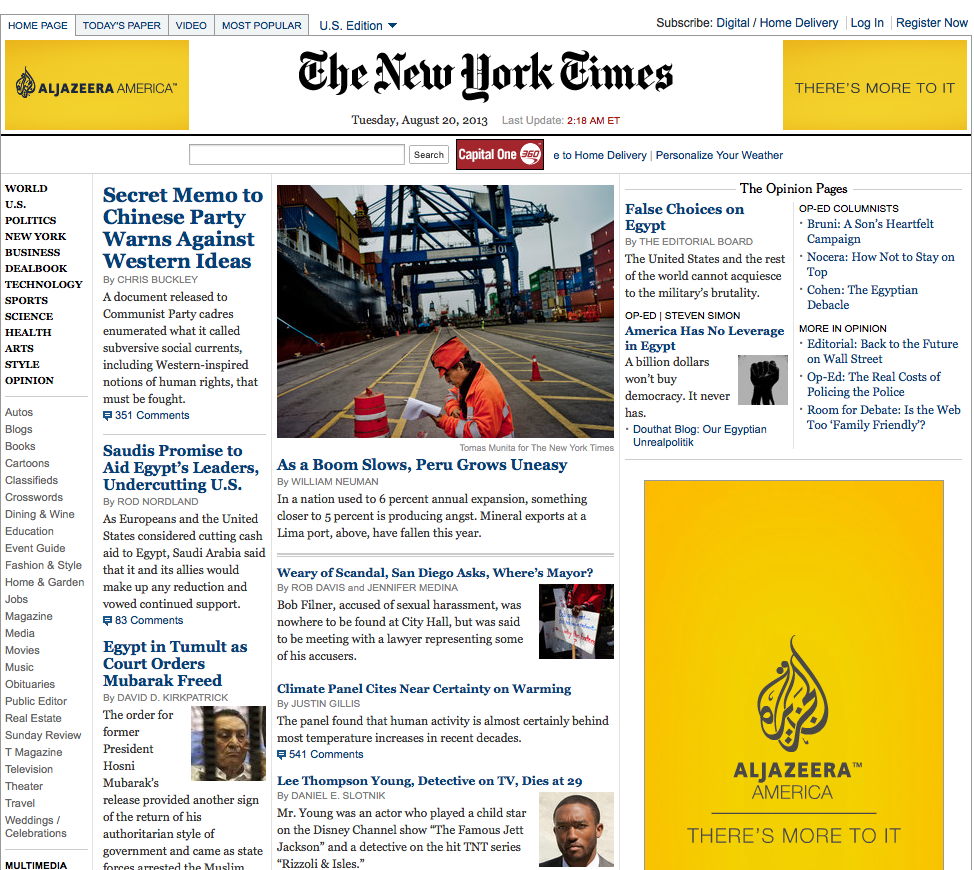This is a screenshot of a computer displaying a webpage for Al Jazeera America, as indicated in the upper left corner within a yellow rectangle. To the left of this label, there is an emblem resembling a fire symbol. 

Centered at the top of the screen is a header reading "The New York Times," followed by the date, "Tuesday, August 20th, 2013." Below this header, several article titles are listed in blue text, accompanied by the article text in black.

The first article in the upper left corner is titled "Secret Memo to Chinese Party Warns Against Western Ideas" by Chris Buckley. This article details a document distributed to Communist Party cadres, enumerating what it describes as subversive social currents, including Western-inspired notions of human rights that must be combated.

The center of the screenshot features a photograph situated below The New York Times header. The image depicts a bustling shipping dock. On the left side, a large container ship is visible, while to the right, there are big rectangular shipping containers. In the foreground stands a worker, clad in an orange jacket and hat, both adorned with reflective tape. He is looking down at a piece of paper. Additionally, a large orange traffic cone is positioned nearby on the road.

The screen showcases several other articles and elements, providing a comprehensive snapshot of the webpage.